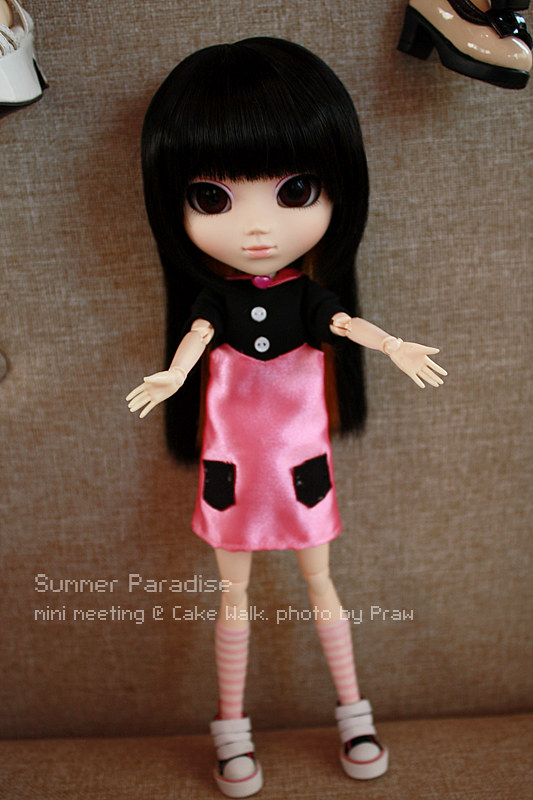In the center of the image, a detailed figurine of a little girl doll stands prominently. The doll, which appears to be Asian with long black hair and big black eyes, is dressed in a pink dress with black borders, featuring black pockets towards the bottom, and white buttons at the top. Her jointed arms are stretched outwards as if calling for a hug, and she is positioned directly at the center of the image. The doll is standing with her legs slightly apart, wearing pink and white striped socks paired with white, pink, and black velcro shoes.

The scene is set against a fabric surface believed to be a brown couch or a similar piece of furniture, extending both at the bottom and as the backdrop of the image. In the upper left and upper right corners, there are hints of additional shoes, likely belonging to other dolls, contributing to the overall atmosphere that suggests an indoor setting–possibly a toy store or a personal collection display.

The image bears a watermark at knee level of the doll, reading "Summer Paradise Mini Meeting and Cakewalk. Photo by Prawl.” The colors in the photograph are predominantly white, tan, brown, black, and pink, enhancing the warm and inviting mood of the scene.